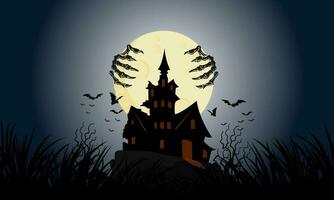This image depicts a spooky, Halloween-esque scene with a dark, shadowy ambiance. Dominating the picture is a large, bright yellow moon centrally positioned against a gray, textured background that fades to black at the edges. Two skeletal hands, appearing gray, grasp the outer sides of the moon, enhancing the eerie effect. Beneath this moon, a foreboding, elaborate house stands, resembling a haunted mansion with sharp architectural features and a prominent tower. The house is rendered in dark hues, its windows and door strikingly highlighted in gold, suggesting light emanating from within. The structure seems perched on a rugged, unkempt hill, with barren, twisted tree branches or twigs emerging from below. Adding to the ominous atmosphere, a flock of black birds or bats flutters around the silhouette of the house. The overall scene, computer-generated and surreal in its presentation, evokes a chilling, nighttime setting, rich in gothic and paranormal elements.